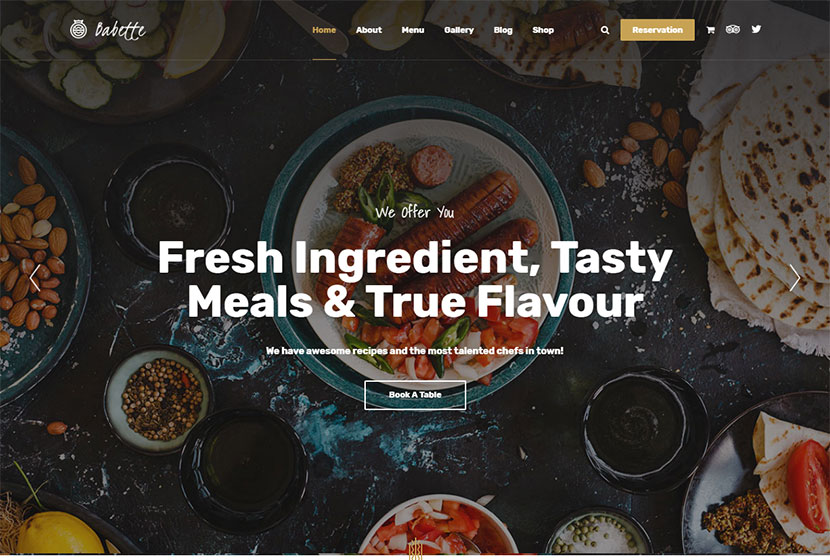The image features a predominantly black background adorned with various pictures of food. On the center left, there are visible almonds, while the top left corner seems to depict some kind of vegetables, though they aren't clearly identifiable. On the lower right side, there are pieces of pita bread garnished with tomatoes and what appears to be ground beef. 

At the heart of the image lies a plate brimming with assorted food items. Above this plate, to the top left, there's an indistinct circular shape with a filled-in box on top of it, accompanied by an illegible word. The central region of the image prominently displays the word "Home" in yellow, followed by "About," "Menu," "Gallery," "Blog," and "Shop" in white text. A magnifying glass icon is also present, alongside a yellow rectangle bearing the word "Reservations."

Further to the right, there appears to be a shopping cart icon, although it is not clearly visible. Next to it are some additional unclear elements, followed by the well-known Twitter bird symbol. Beneath these elements, a white text overlay declares: "We offer you fresh ingredients, tasty meals, and true flavor. We have awesome recipes and the most talented chefs in town."

Additionally, there is a white-outlined rectangle containing the text "Book a Table," inviting viewers to make a reservation.